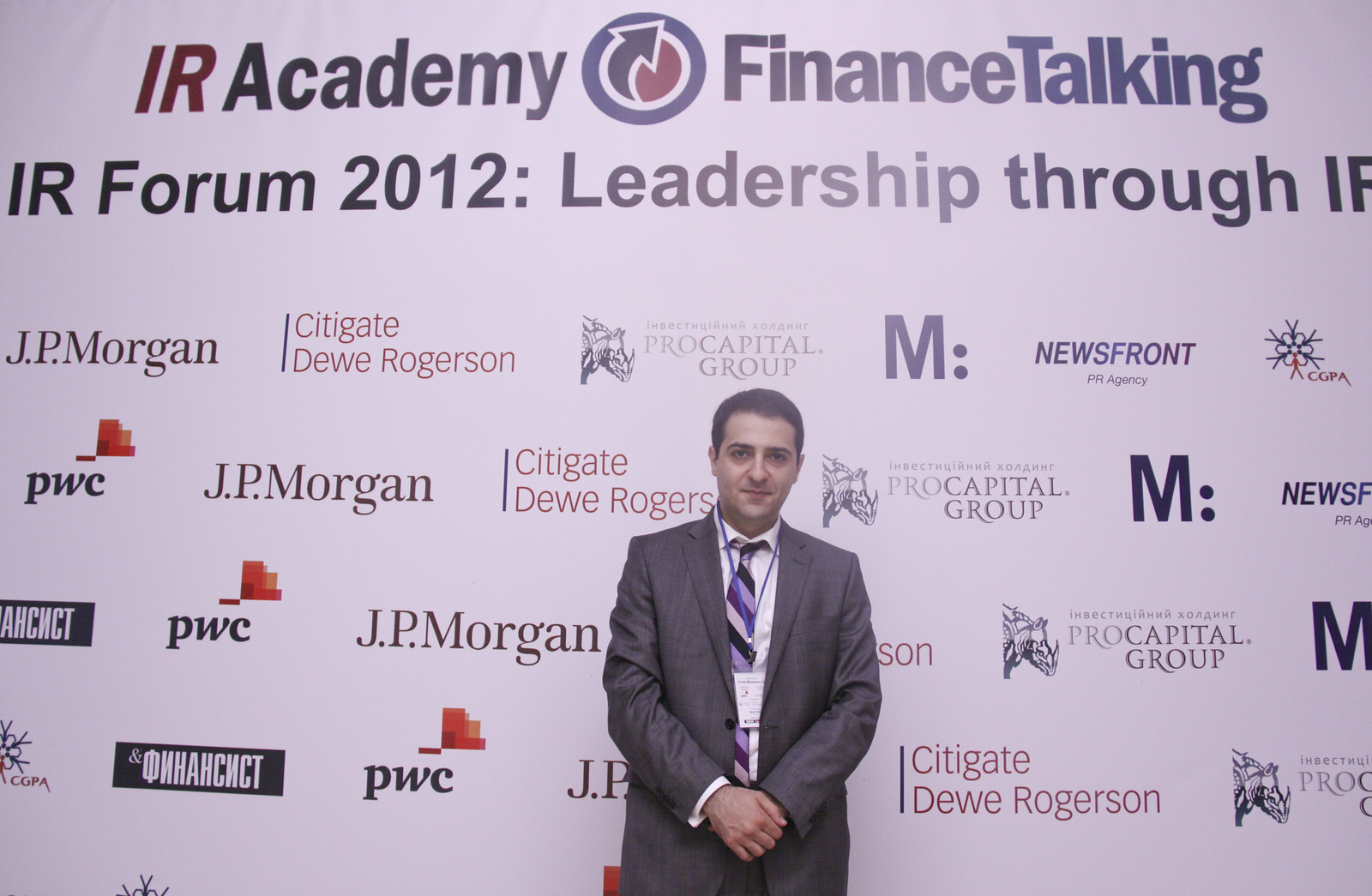This photograph features a man with short, dark hair and an olive complexion, standing confidently in front of a large, wall-sized poster. He is dressed in a gray business suit, a white button-down shirt, and a striped tie in blue, black, and white hues. An ID badge hangs from a lanyard around his neck, and his hands are folded neatly in front of him as he looks at the camera with a composed expression.

The backdrop prominently displays the text "IR Academy" at the top, followed by "Finance Talking" and "IR Forum 2012: Leadership through IP" (though part of this last line appears to be cut off). A distinct logo, comprised of a blue circle with a red half-circle and an upward-facing arrow, is also featured. Below the main title, various sponsors are listed, including notable names such as JPMorgan, CityGate, Dew, Rogerson, PwC, Pro Capital Group, and News Front, with at least one sponsor's name written in Russian letters. The sophisticated yet simple backdrop places the man front and center, suggesting his participation in a significant conference or forum.